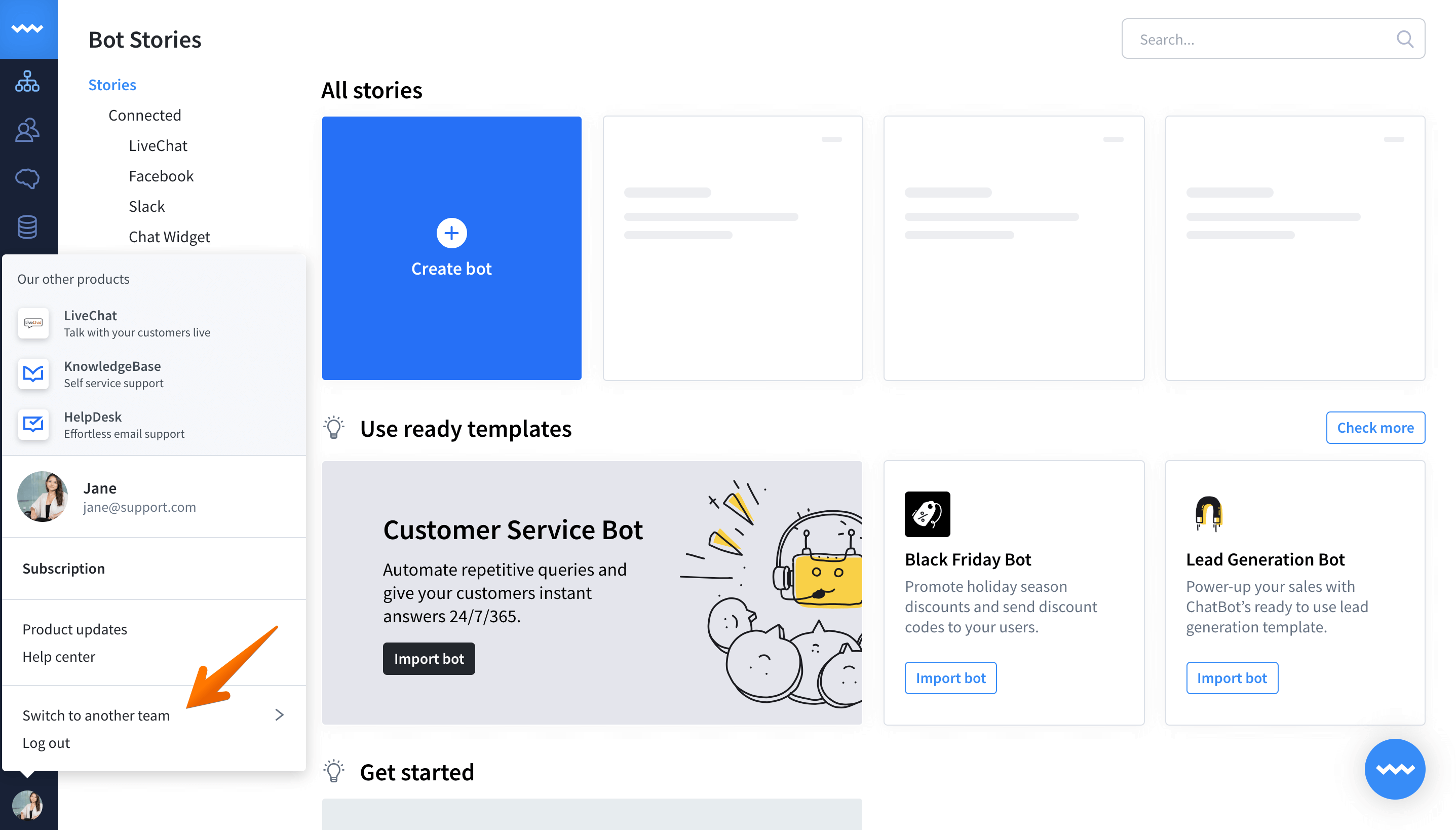In this image, we see a detailed screenshot of a support service interface page. The page contains various text elements including options such as "Stories," "We have connected," "Live Chat," along with icons for Facebook, Slack, and Chat Widgets. The interface also showcases the segment "Our Other Products" under which options like "Live Chats," "Talk With Your Customers," "Knowledge Base," and "Self-Service Support" are listed, emphasizing different assistance solutions such as "Help Desk" and "Effortless Email Support."

In the profile section, we see the user "Jane" associated with the email address support@example.com. Additional options available include "Subscription," "Product Updates," "Help Center," and "Switch to Another Team," with an arrow pointing to this option located towards the bottom left corner of the image. The "Logout" button is also visible.

The interface highlights customer service automation, showcasing "Customer Service Bots," which aim to automate repetitive queries and provide instant answers to customers. Other bot options displayed include "Black Friday Bots" and "Lead Generation Bots," along with an option to "Create a Bot." Finally, text indicating "Support 24/7, 365" (likely meant to convey round-the-clock support) is also prominently displayed.